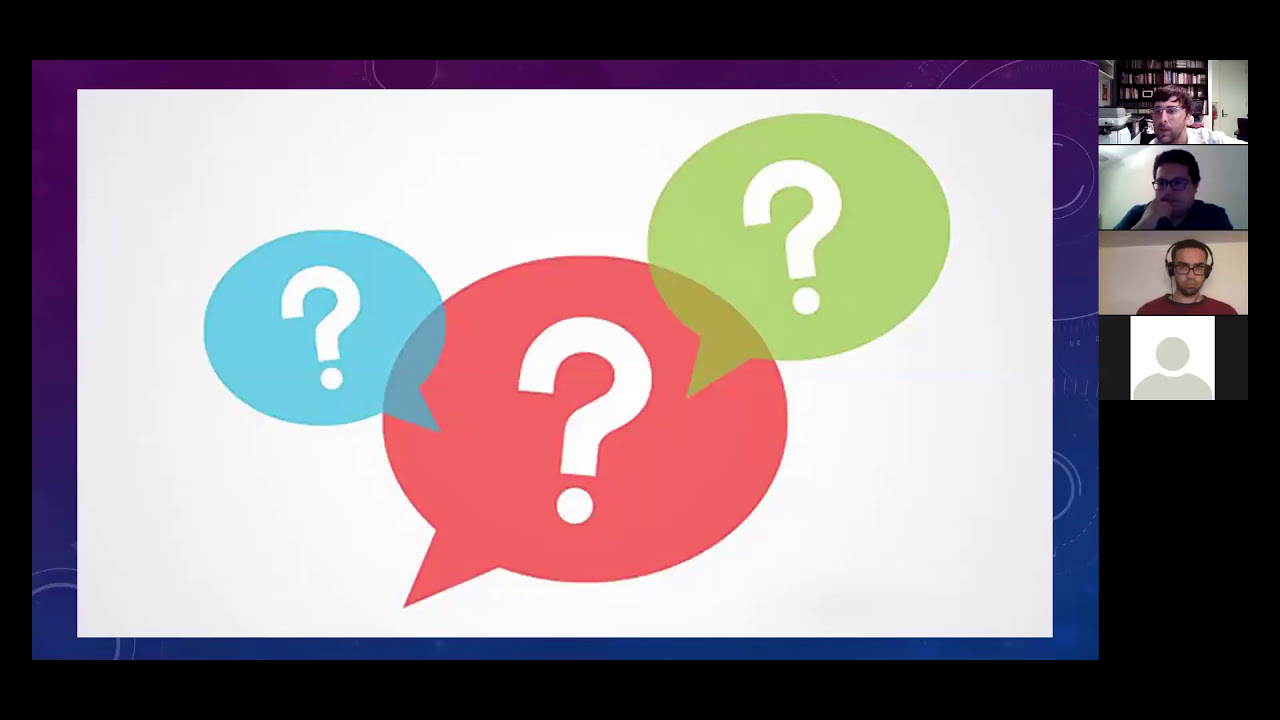This image is a detailed screenshot from an online video conference call, incorporating both digital animation and hyper-realistic, faux-rough elements. Occupying the leftmost three-quarters of the screen is the primary shared content, which presents a large white box framed by a purple and blue border. Inside this two-dimensional box are several overlapping clipart speech bubbles, each containing a white question mark. The central speech bubble is red, flanked to the right by slightly smaller green and blue bubbles, both also featuring white question marks.

The right quarter of the screen displays a sequence of five small panels. The topmost panel shows a Caucasian man with brown hair and thin-framed glasses, sitting in a room with a bookcase behind him. Below him, another man with dark hair and glasses sits in front of a plain white background, followed by a brown-skinned man wearing black headphones and a red shirt, also against a white backdrop. The final visible panel shows a grayscale cartoon avatar, indicating a participant who has opted not to display their image. The last panel at the bottom is just black. This meticulously detailed scene appears to capture the essence of a collaborative presentation or discussion during the video call.